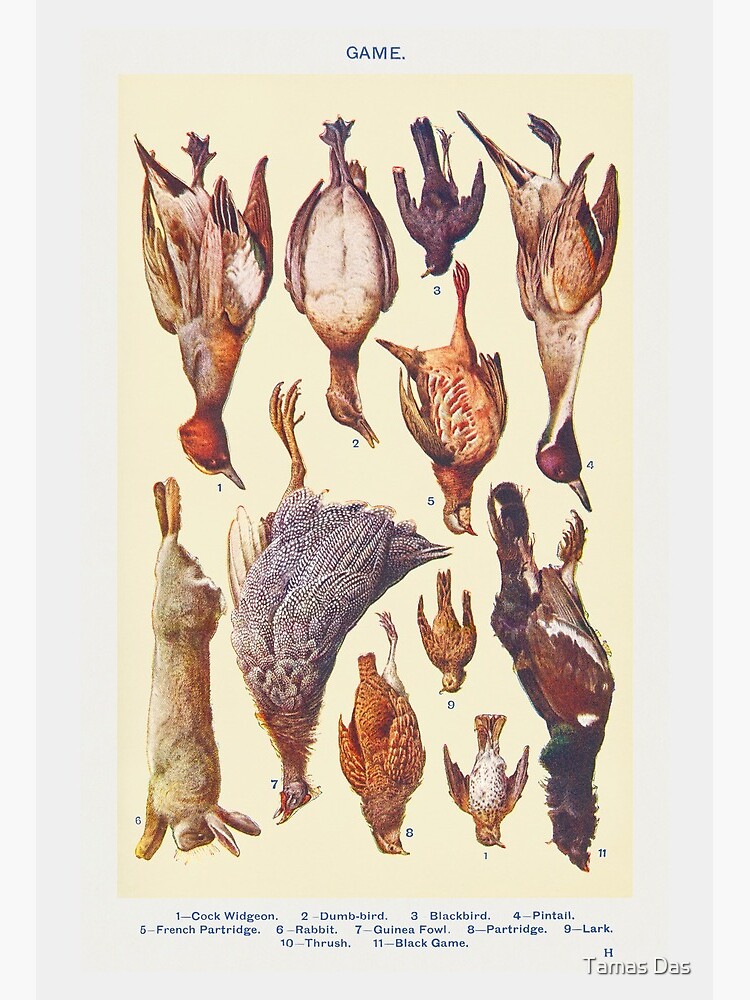This is a detailed illustration that appears to be from a book, showcasing an array of game animals hanging upside down as if freshly caught. The image is vertically oriented, framed with a gray border, and features a dull yellow background. At the top, the word "Game" is prominently displayed, indicating the theme of the illustration. There are 11 different animals depicted, primarily birds, each meticulously labeled with a number and corresponding descriptor listed at the bottom of the image. The animals include:
1. Cockwidgeon
2. Dumbbird
3. Blackbird
4. Pintail
5. French Partridge
6. Rabbit
7. Guinea Fowl
8. Partridge
9. Lark
10. Thrush
11. Black Game.

These animals are illustrated in a lifelike and detailed manner, suggesting they have been hung post-capture before dressing. The image also includes the name "Thomas Das" at the bottom, potentially indicating the artist or author.